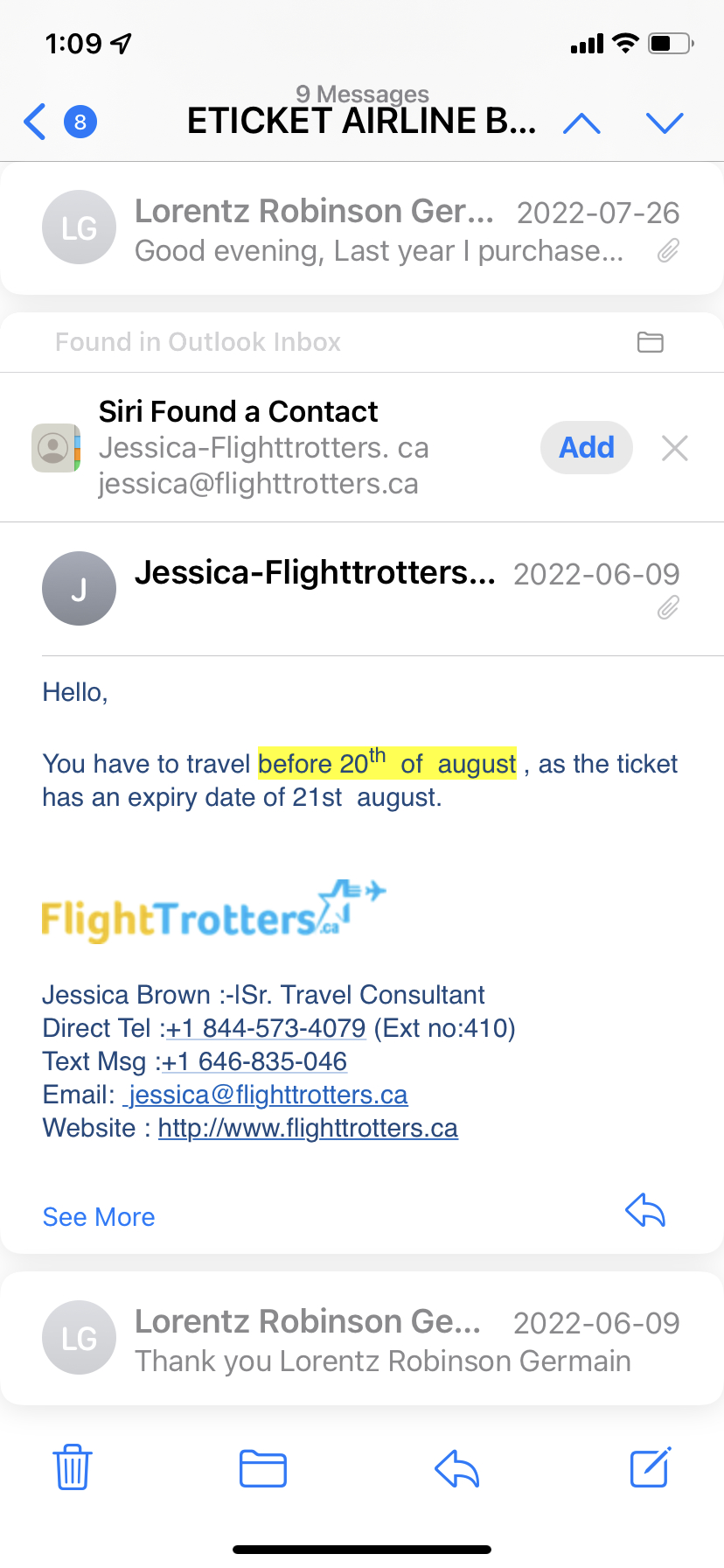This image is a screenshot from a mobile email application, likely Apple's Mail app judging by its light white interface and the layout. At the top of the screen, it indicates that there are "9 messages" and specifically highlights a category labeled "e-ticket airline." The visible list of emails pertains to e-ticket airline communication, with the topmost message from Lorenz Robinson dated July 26, 2022. 

Beneath that, there's an automatic suggestion stating "Siri found a contact, Jessica-Flighttrotters.ca." Further down, an email from Jessica-Flighttrotters, dated June 9, 2022, is open. This email advises that travel should be completed before August 20th, as the ticket will expire on August 21st. The signature at the end of the email features the Flighttrotters logo, which is yellow and blue, and includes the sender's details: "Jessica Brown, Senior Travel Consultant," along with her contact information.

At the bottom of the screenshot, there are several icons representing different actions within the app, including options to delete (trash button), organize (folders button), and compose a new email (create new email button).